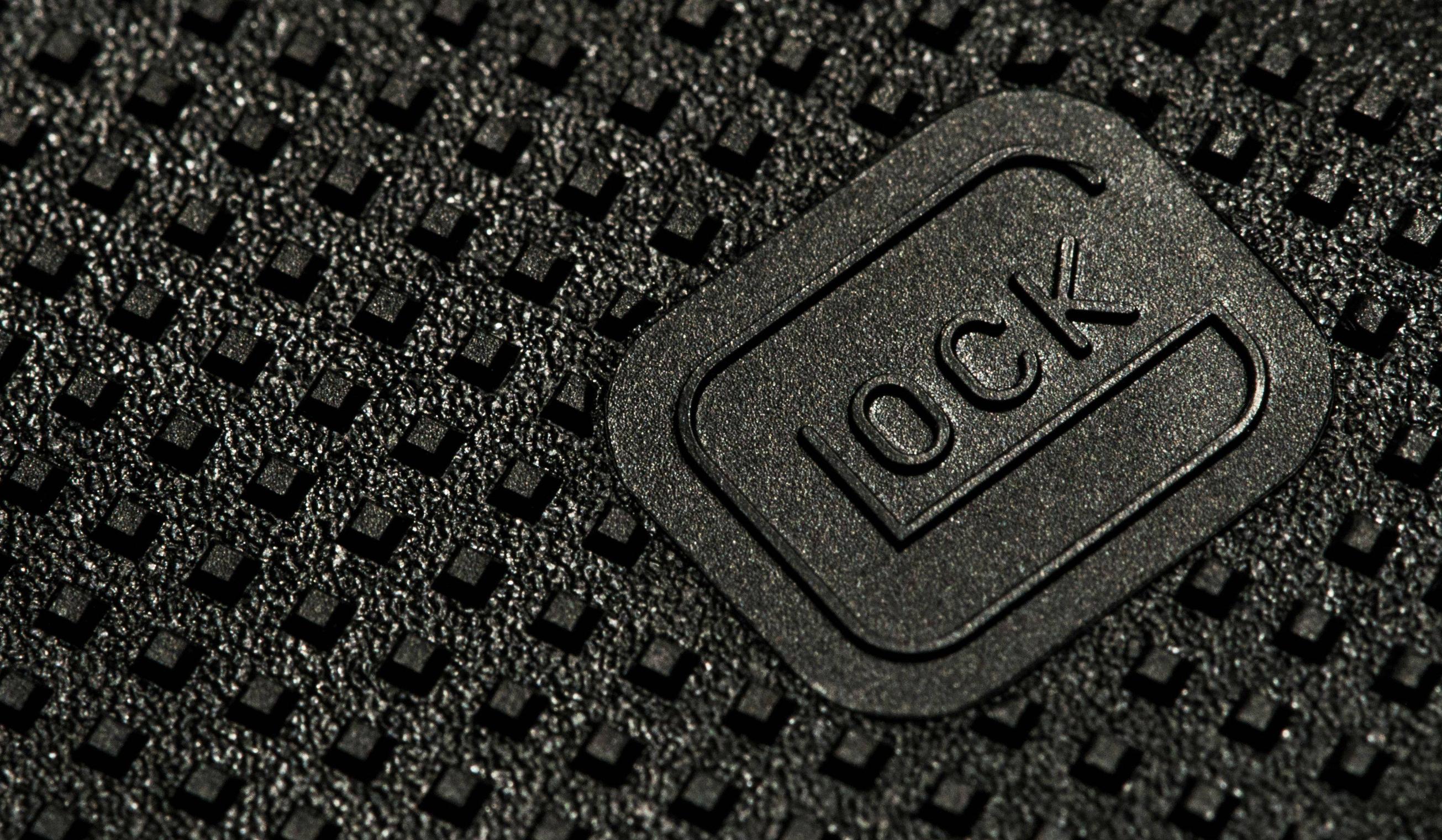This highly magnified image shows a detailed view of a black textured material, possibly metal, rubber, or plastic. The surface features a grid of small, evenly spaced half-cube bumps that create a grainy texture, interspersed with reflective spots that catch the light, appearing as tiny white specks. Prominently on the right side of the image, there is a smooth, rounded rectangular button embedded within this bumpy background. The button bears a distinctive logo that includes what appears to be the word "LOCK" or "OCK," integrated into a design resembling a 'G' shape with an upward-pointing line. This image likely depicts an object such as a lock button from a car's interior door handle.